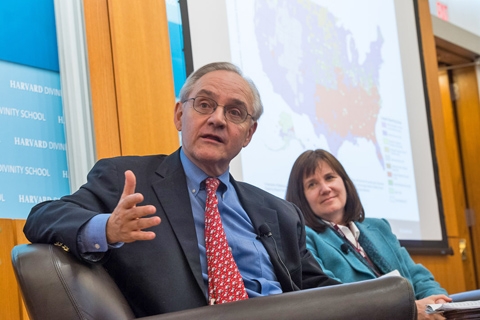The photograph features an older gentleman and a woman seated on a black leather couch. The man, who is wearing a dark suit jacket, a medium blue shirt, and a red tie with a white design, has his right hand stretched out towards the camera as if he is making a point while speaking. He is also wearing spectacles and has a microphone clipped to his left lapel. Next to him, the woman with dark brown shoulder-length hair, slight bangs on her forehead, and a turquoise jacket, attentively looks at him. She too has a microphone on her lapel and a scarf around her neck. Behind them, a large screen displays a map of the United States, and to the right side of the image, there is a yellow doorway.